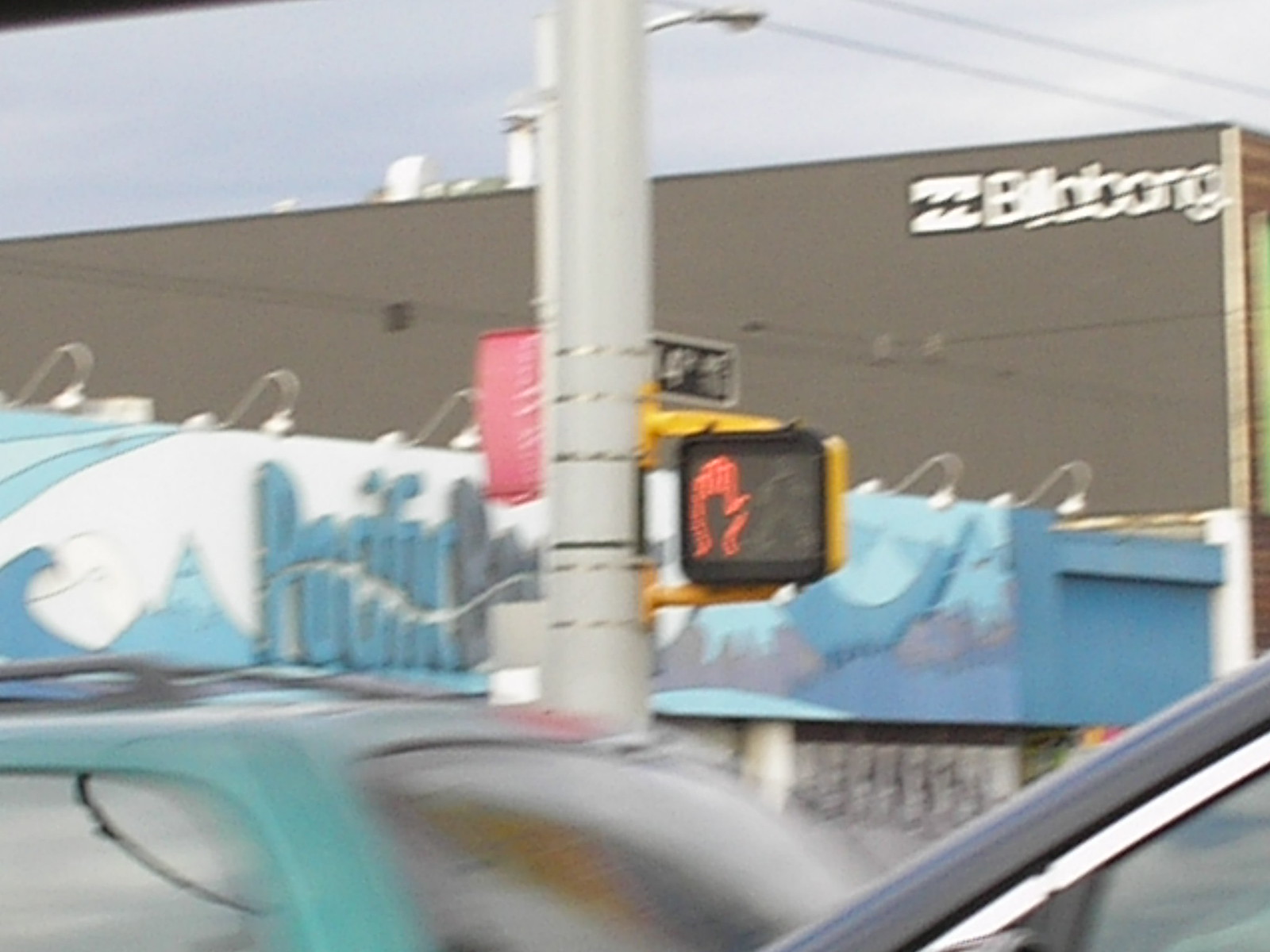This color photograph captures an urban street scene with a variety of elements. Dominating the background is a tall, brown building with the brand name "Billabong" clearly visible in white lettering at the top right corner. In the center of the image, partially obscured by a large gray lamppost, is a portion of a blue building with the word "Pacific" visible. Affixed to the lamppost is a pedestrian crossing sign, which displays a red stop hand indicating it is not safe to cross. Overhead, the sky is overcast and gray, adding a muted tone to the scene. At the bottom of the image, two vehicles are partially visible; the one on the left is turquoise, while the one on the right is gray. Due to their incomplete presence in the frame, the specific types of these vehicles remain unclear.